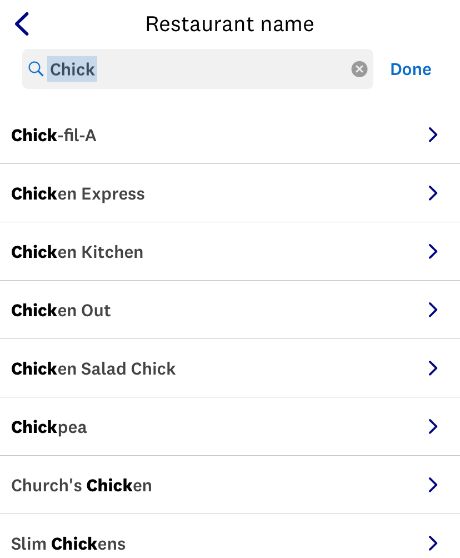The image captures a search interface, likely from a restaurant-finding app or website. In the top left corner, a blue arrow points left, adjacent to a dark gray text reading "Restaurant Name." Below this title, a search box features a magnifying glass icon, indicating a search function. Within the search box resides the input "CHICK." To the right of this input field is a "Done" button, suggesting that the user has finished typing.

Beneath the search box, a list of search results appears, generated from the keyword "CHICK." The top result is "CHICK-FIL-A," followed by "CHICK-EXPRESS," "CHICKEN-KITCHEN," "CHICKEN-OUT," "CHICKEN-SALAD-CHICK," "CHICK-P," "CHURCHES-CHICKEN," and lastly "SLIM-CHICKENS." In each of these listings, the word "CHICK" is highlighted in bold, with the remaining text displayed in a lighter gray font. Accompanying each restaurant name is a rightward-pointing arrow button, indicating that users can click on these results to access more information about the respective restaurants.